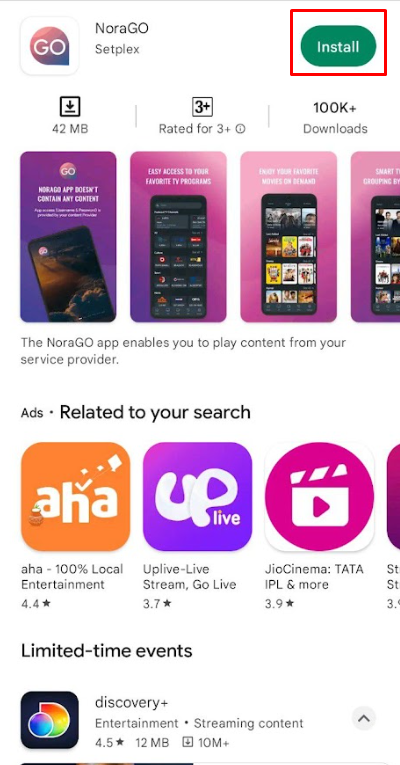"Screenshot of the NORAGO app details page:

The upper section prominently features the app's logo, which consists of the letters 'G' and 'O' within a thought bubble-shaped design on a pink background. To the right of the logo, there's a green Install button highlighted by a red box.

Below the logo and Install button, the page displays a series of four screenshots that showcase different functionalities of the NORAGO app. These images illustrate the app being used on a smartphone. Key information about the app is provided, including:
- App size: 42 megabytes
- Suitable for ages 3 and up
- Over 100,000 downloads

The description indicates that the NORAGO app allows users to play content from their service provider. This is followed by a section titled 'Ads related to your search,' featuring several other apps such as AHA, Uplive Live, and Jio Cinema Tata. 

Further down, information about limited-time events and additional apps like Discovery Plus is provided, which offers entertainment and streaming content. Another highlighted app details section includes:
- Rating: 4.5 stars
- Size: 12 megabytes
- Over 10 million downloads

This screenshot encapsulates the comprehensive information that users are presented with when they search for and click on the NORAGO app, including its features, related apps, and download statistics."